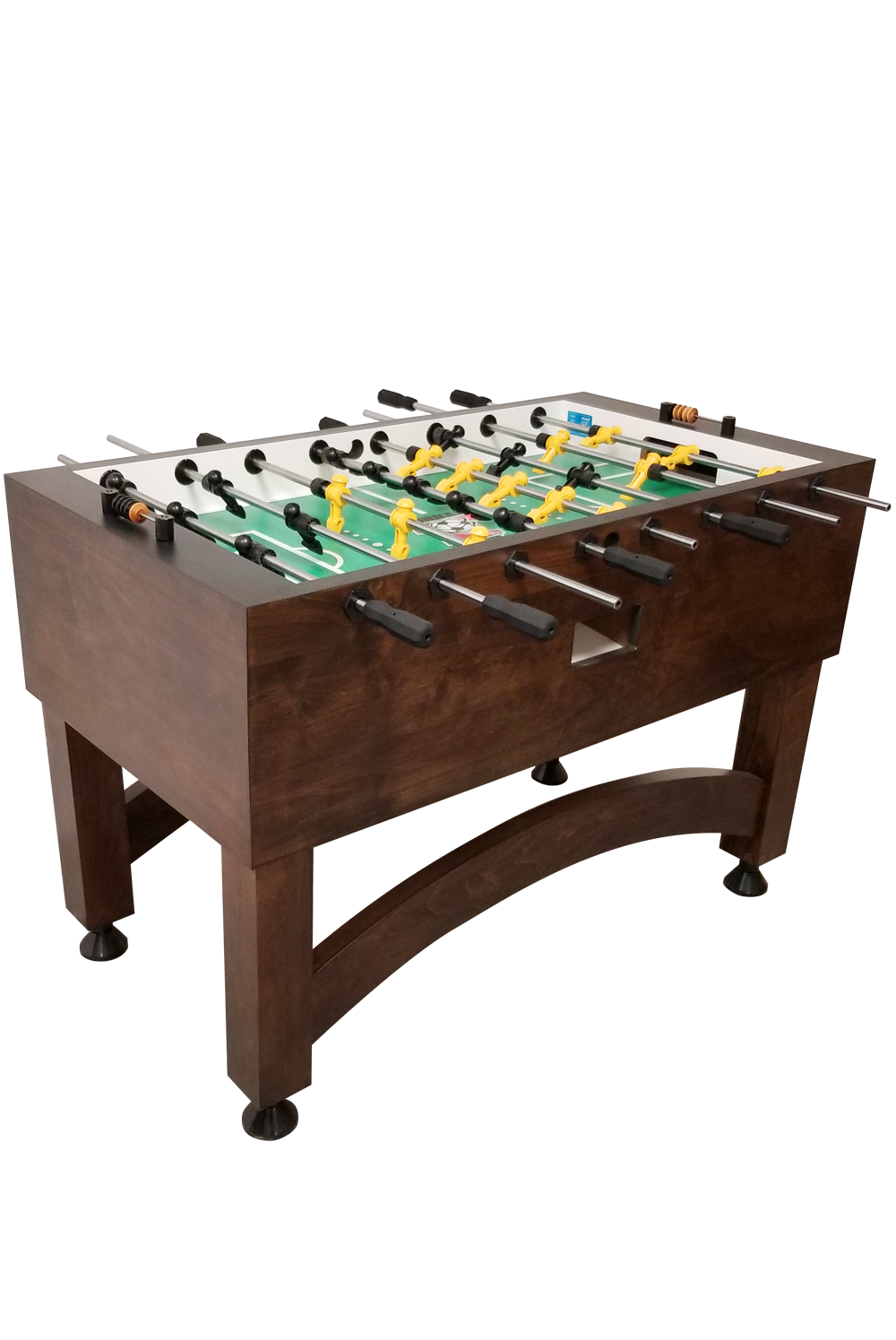This image features a beautifully crafted foosball table with a rich, dark wood finish. The table's sturdy build includes a shiny, curved arch that stretches horizontally between the front and rear legs, enhancing its elegant design. Each leg stands on small, round pegs, ensuring stability. The table showcases two teams of foosball players, one dressed in yellow and the other in black, mounted on sleek silver rods with brown handles. The playing field mimics a soccer pitch, complete with goal areas where players aim to score. The top of the table features discs for tracking scores. Overall, this foosball table is a well-made, visually appealing game set, perfect for enthusiasts.